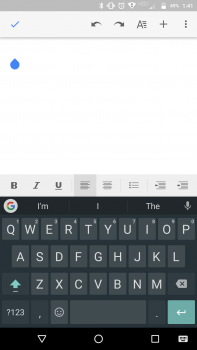This vertically oriented image, resembling a screenshot from a smartphone, presents a detailed view of a typical mobile interface. The top section features a long, dark gray rectangular bar displaying essential status icons centered in white, such as the Bluetooth symbol, battery life indicator, and the current time. Below this, a lighter gray bar contains several icons, starting with a blue check mark on the upper left. Moving right, it includes two dark gray arrows pointing in opposite directions, a large "A" with surrounding lines, a plus sign, and three vertical dots for additional options.

The main portion of the screen is predominantly white, featuring only a single blue raindrop-like icon. Below this area lies another gray strip equipped for text formatting, with options for bold, italicized, and underlined text. The position for inserting text is indicated, with the first option already selected.

At the bottom of the screen is the virtual keyboard, showcasing typical features: dark gray keys with white lettering, the Google symbol, a space bar, predictive text suggestions such as "I'm", "I", or "the", and a microphone icon for voice input. Concluding the image, a black rectangular strip at the very bottom houses three iconic navigation buttons in white: a triangle, a circle, and a square.